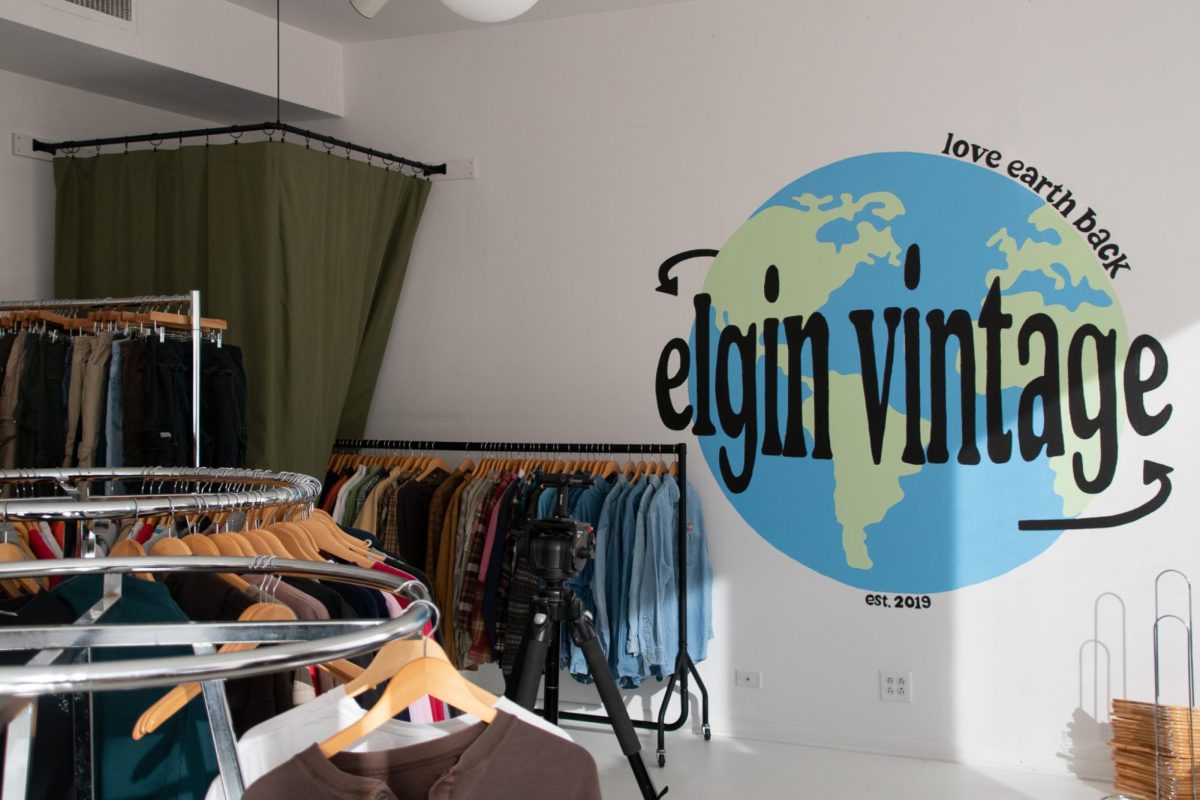This image captures a detailed view of a corner inside a clothing store called Elgin Vintage. The scene is set against light gray walls that meet at a corner on the left side. A green curtain functions as a makeshift dressing room, descending from the top left corner and disappearing behind a collection of clothing. The left half of the frame features an assortment of clothes, including two circular racks densely packed with shirts and a straight black rack against the left wall. Further to the right, another black rack holds pants or shorts. 

Prominently displayed on the right wall is a striking artwork of the Earth, rendered in vivid blue with clearly distinguishable continents. Above this globe, the slogan "Love Earth Back" is inscribed, while the middle bears the store's name, "Elgin Vintage," and its establishment date, "October 2019." Below the globe, a light socket is visible. The bottom right corner of the image shows a stack of brown paper bags or similar items, neatly placed in a metal holder. Overhead, a vent is visible at the top left corner of the ceiling, and a white hanging light illuminates the room.